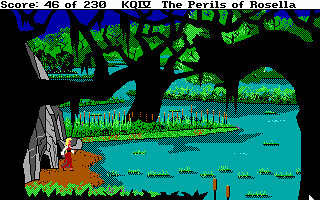A vintage computer game screenshot depicts a scene from "The Perils of Rosella." The graphics are visibly pixelated, indicative of an older game era. At the top of the screen, text displays a score of 46 out of 230 and includes some characters from an unfamiliar language. Central to the image, a woman with long blonde hair, presumably Rosella, stands on a dirt patch as if she has just emerged from a cave embedded in a rock face. Surrounding her is a murky, swamp-like pond adorned with green plants. Black silhouetted trees with bare branches protrude from the water, enhancing the eerie atmosphere. In the distance, more trees with lush green foliage contrast the desolate foreground.